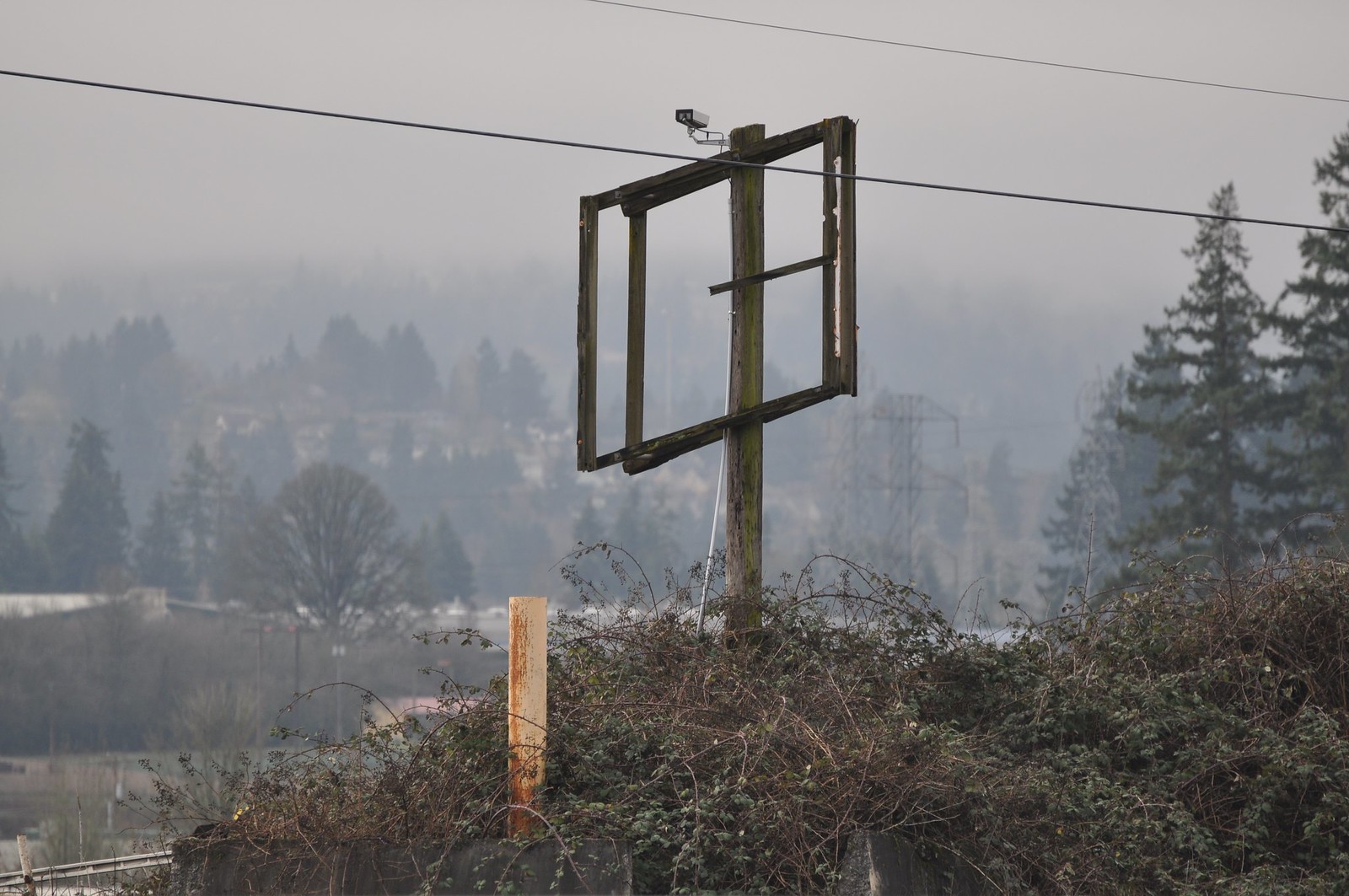The photograph captures a somber outdoor scene on a dark winter day. In the foreground, you can see several old trees, some possibly dead or dormant due to the cold season, displaying a mix of lingering green and dominant brown foliage. Emerging from these trees is a brown pole, and nearby, a larger rectangular signpost, now empty and devoid of signage, suggests that a business may have once operated in this location. Mounted atop this vacant signpost is a sleek, long gray and black security camera. Spanning horizontally across the image are extended electrical lines, with the background revealing a backdrop of towering pine trees and tall electrical poles. A light dusting of snow covers parts of the scene, enhancing the wintery atmosphere.